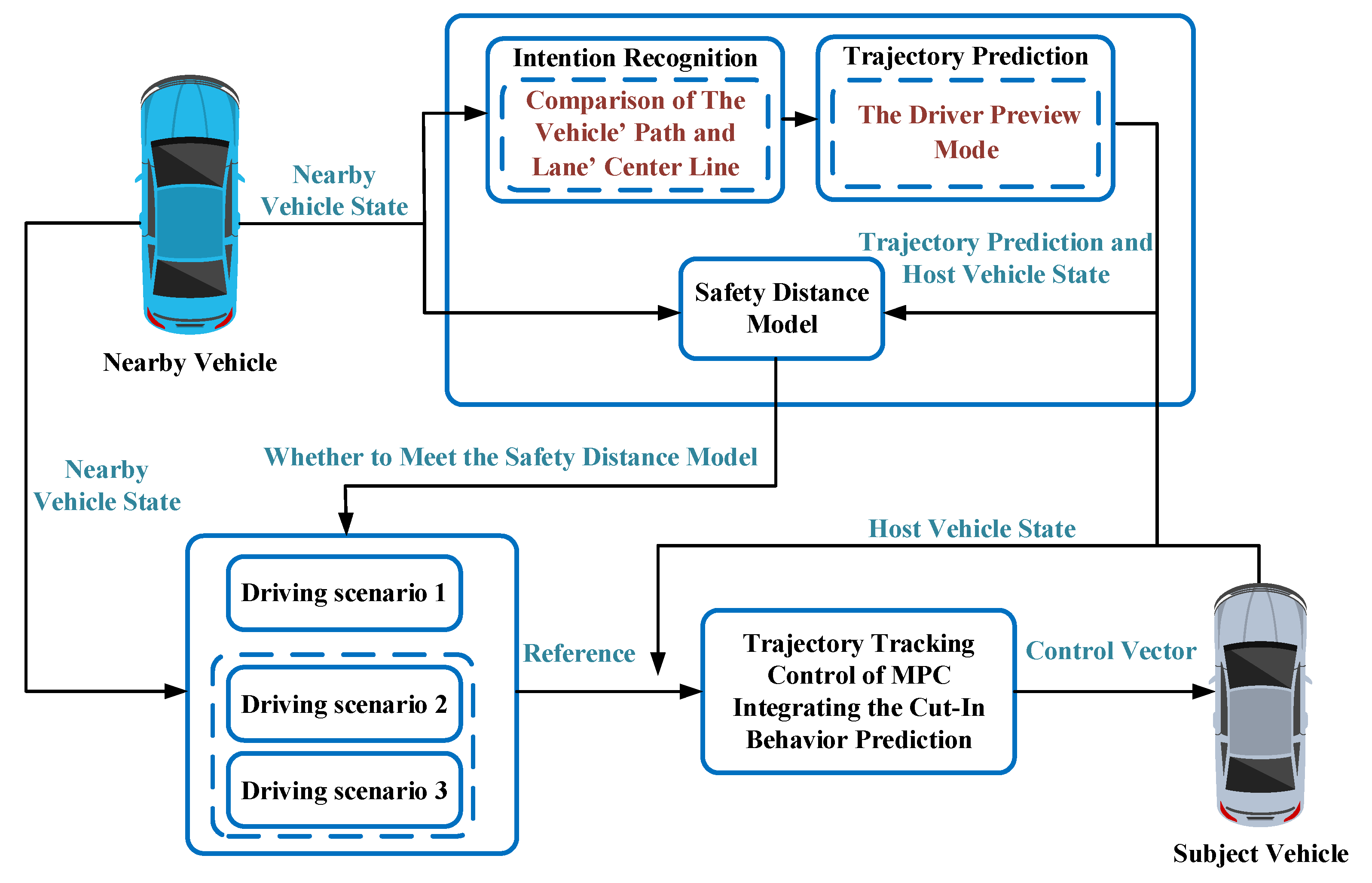The image depicts a comprehensive diagram related to vehicle behavior prediction and control. On the top left, a top-view drawing of a blue car is labeled "Nearby Vehicle," and it forms part of a complex flow chart. This section includes angular black and blue lines or squares, with a surrounding black line and blue boxes containing terms such as "Intention Recognition," "Comparison of the Vehicle Path," "Center Lane," "Trajectory Prediction," "The Driver Preview Mode," and "Safety Distance Model."

In contrast, the bottom right features a grayish car labeled "Subject Vehicle," with an arrow pointing toward it labeled "Control Vector." Adjacent to this, another blue box is labeled "Trajectory Tracking Control of MPC" and includes "Integrating the Cut-In Behavior Prediction."

The diagram as a whole connects various scenarios, including "Driving Scenario 1, 2, and 3," and illustrates relationships between different vehicle states and prediction models, including safety and trajectory control mechanisms.